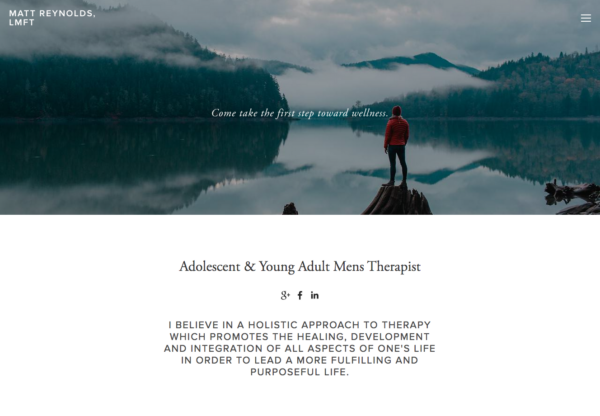Website for a Therapist:

The website features a prominent header image depicting a serene lake with trees on the distant shore partially engulfed by a delicate fog that also covers the hills. In the foreground, a person stands on a jutting piece of land, symbolizing contemplation and the journey toward wellness. Overlaid on this tranquil scene is the text: "Come Take the First Step Towards Wellness." In the upper left-hand corner, the therapist's name, "Matt Reynolds, LMFT," is displayed, while the upper right-hand corner features a hamburger menu icon. 

Below the header, on a clean white background, the text reads: "Adolescent and Young Adult Men's Therapist." This section also includes logos for Google Plus, Facebook, and LinkedIn, indicating social media connectivity. Additionally, a statement from the therapist emphasizes a holistic approach to therapy: "I believe in a holistic approach to therapy which promotes the healing, development, and integration of all aspects of one's life in order to lead a more fulfilling and purposeful life."